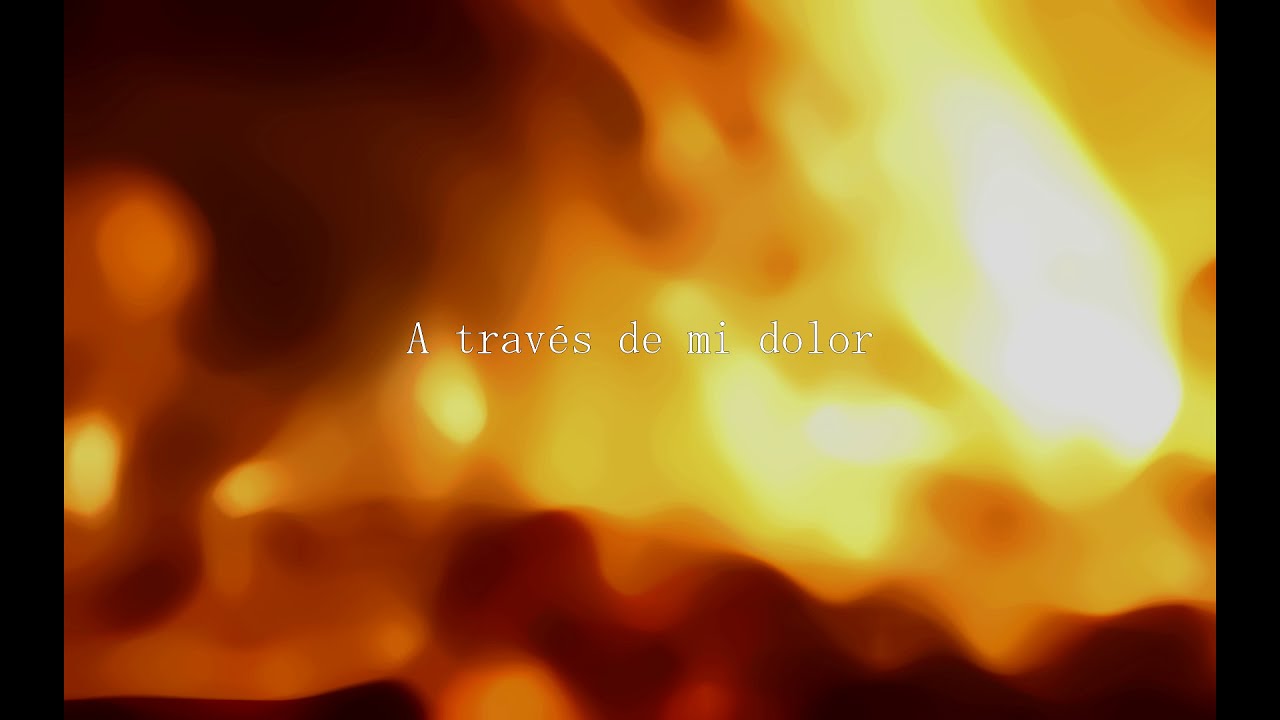The image features a blurred, fiery background with an array of colors that evoke the intense hues of a flame, such as deep yellows, intense oranges, dark reds, and maroons. The background, possibly depicting a campfire or fireplace, gives a sense of warmth and movement, appearing wavy and intentionally out of focus to enhance the artistic effect. Dominated by colors of brown, yellow, orange, and occasional black sections, the scene includes both vertical black strips on the sides, adding to its captivating composition. In the center of the image, there is a text in white capital letters, "A TRAVES DE MI DOLOR," which appears to be in Spanish, translating to "Through My Pain." This mix of vivid colors and evocative text suggests a powerful blend of visual and emotional elements, possibly as a screenshot from a film or a digital artwork.